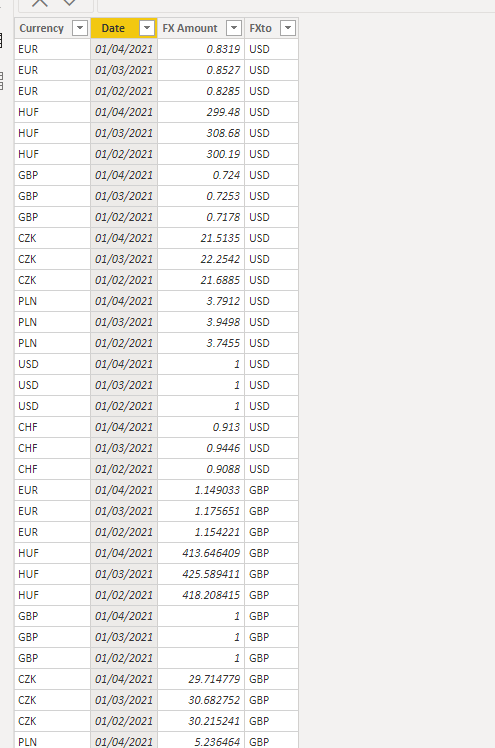The image is a detailed screenshot of a spreadsheet with a gray background, likely from a computer program. The spreadsheet contains four columns labeled, from left to right: "Currency," "Date," "FX Amount," and "FXTO," each marked with a downward arrow indicating sortability. The "Date" column is highlighted in yellow, emphasizing its active status, while the other column headers are in gray. 

Coded in white and gray alternating rows, the "Currency" column lists various currency abbreviations including EUR (Euros), HUF (Hungarian Forint), GBP (British Pound), CZK (Czech Koruna), PLN (Polish Zloty), USD (US Dollar), and CHF (Swiss Franc). This sequence repeats multiple times. The "Date" column features dates clustered around early January 2021, specifically ranging from the second to the third of January. Both the "FX Amount" and "FXTO" columns contain placeholder data represented by white blocks, maintaining a clean, structured appearance. The image spans more than half the screen, showcasing a thorough enumeration of data entries while retaining a professional and organized layout.